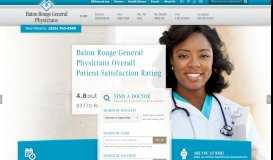The image is a blurry screen capture of what appears to be a medical website. At the top, there's a thin teal border, followed by white sub-menus, which are indiscernible due to the poor quality. A possible search box is also present. Below this, there is a light gray tab with black font, a teal and white logo, and accompanying sub-menus in gray.

The main focus of the image is a smiling African American doctor, wearing a white coat and a stethoscope around her neck. Adjacent to her head, a white box with teal font seems to convey general information, potentially including a patient satisfaction rating, likely 4.8, although it's too blurry to confirm.

Further down, there's another box in off-white and teal, featuring a gray magnifying glass icon and text fields. At the bottom, a teal section contains white icons resembling a calendar and a watch, flanked by a gray scroll bar.